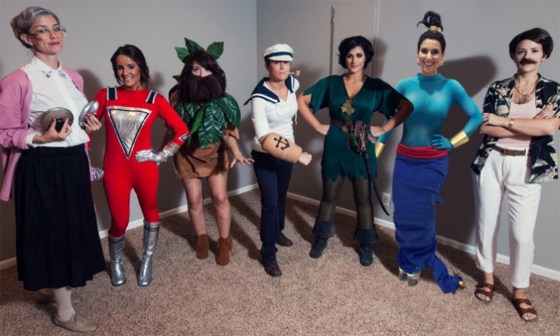The photograph captures a group of seven young women standing in a carpeted room with gray walls, each dressed up as a different Robin Williams character for Halloween. Starting from the left, the first woman is dressed as Mrs. Doubtfire, complete with a long black skirt, a white shirt, her hair in a bun, and holding two pan lids at her chest. Next to her is Mork from "Mork and Mindy," wearing a red suit with silver gloves and striking a confident pose with her hand on her hip. Following Mork is a woman dressed as Alan Parrish from "Jumanji," featuring a rugged look with leaf attire and a large beard. The fourth costume is Popeye the Sailor Man, distinct with the iconic sailor hat and pipe. Next, a lively portrayal of Peter Pan, sporting a green outfit, brown shoes, and a sword. Sixth in line is the Genie from "Aladdin," garbed in vibrant colors, bringing a touch of magic to the group. Finally, on the far right stands a woman dressed as Armand Goldman from "The Birdcage," wearing a floral shirt, white pants, sandals, and a big mustache. The overall ambiance of the photo is somewhat surreal, with the lighting and arrangement giving the characters a cutout-like appearance. Despite the room's muted colors, the costumes provide a burst of reds, blues, greens, and other bright hues, embodying an evening of fun and nostalgia.